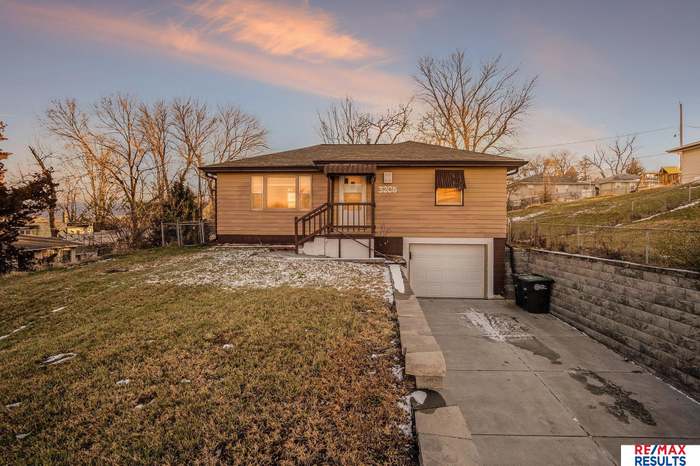In this horizontal rectangular photograph of a split-level suburban house, a "REMAX Results" sign in the lower right corner suggests the property is for sale. The home, featuring brown siding and complementing brown roof and trim, includes a single-car basement garage with a white roll-up door. The concrete driveway leading to the garage is flanked by retaining walls; the left wall is notably tall due to the hillside terrain. 

Above the garage, a single window provides light to the rooms inside. To the left of the garage is a small entrance porch accessed via a flight of stairs. Adjacent to this entrance is a large living room window divided into three sections. The home's front yard stretches above the left retaining wall, showcasing green grass and a dusting of snow hinting at winter. The clear day with blue skies and some white clouds adds to the appeal, while leafless trees in the backyard and neighboring properties indicate the season. The fenced backyard can be seen in the background, providing a sense of privacy and space. Garbage cans are visible near the garage door, emphasizing the functionality and practicality of the home.